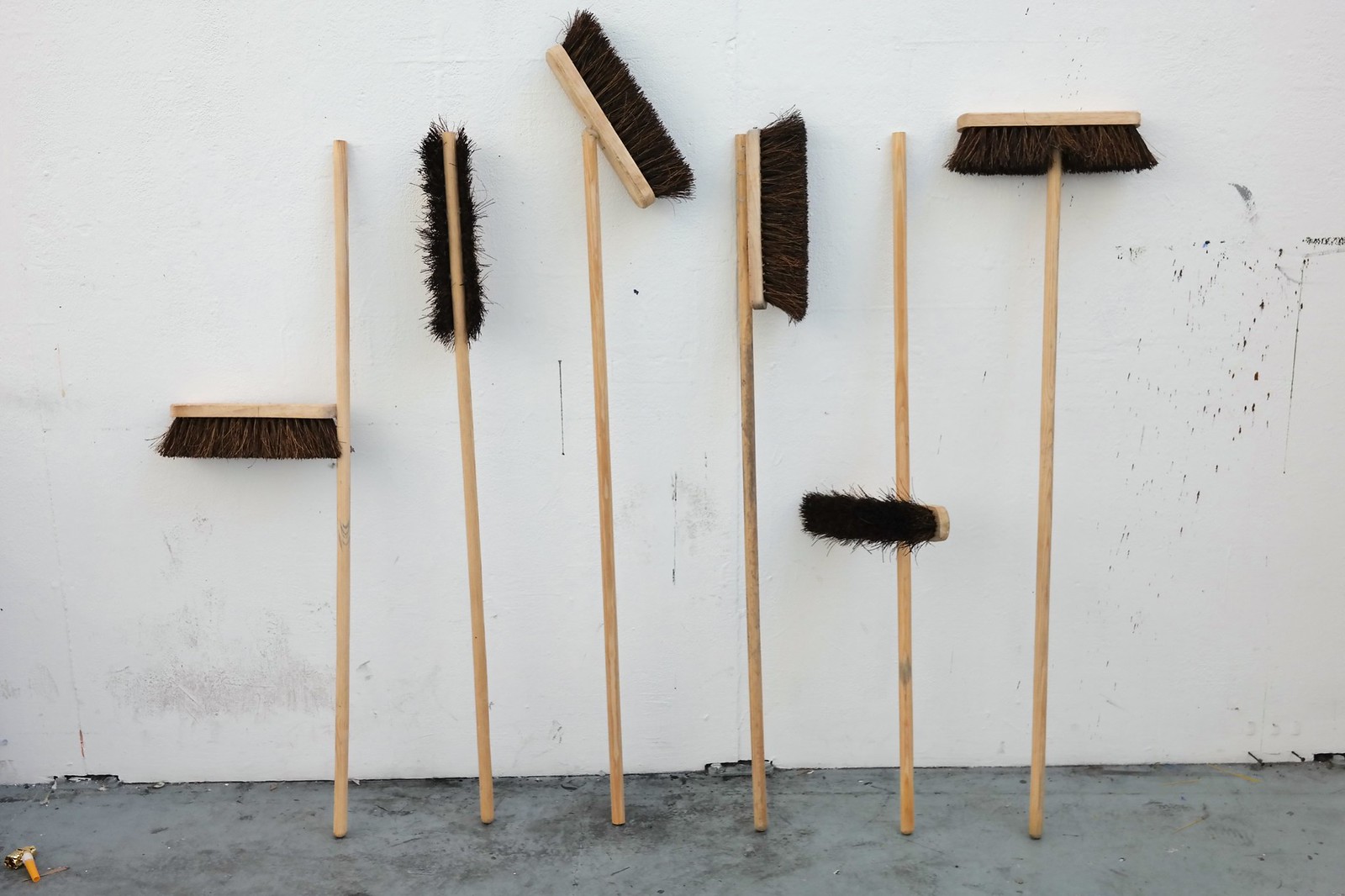The photograph depicts six long wooden brooms, each with a brown handle, leaning against a light gray wall marred by tiny black paint splashes. The uneven, dark gray cement floor adds to the backdrop. The first broomstick on the left stands straight up, with its black bristle head unattached and suspended midway down the handle, leaning against the wall. The second broom's bristle head is vertically behind the handle against the wall, with the bristles facing outward. The third broom's bristle head tilts diagonally from the top of the handle downwards. The fourth broom resembles a toothbrush with its bristle head attached straight on top, pointing rightwards. The fifth broom has its bristle head secured horizontally about one-quarter from the bottom, facing left. The sixth and final broom's bristle head rests atop the handle, resembling a hat or mustache with the bristles pointing downward. Notably, an orange-handled brush with gold bristles lies in the bottom left corner.